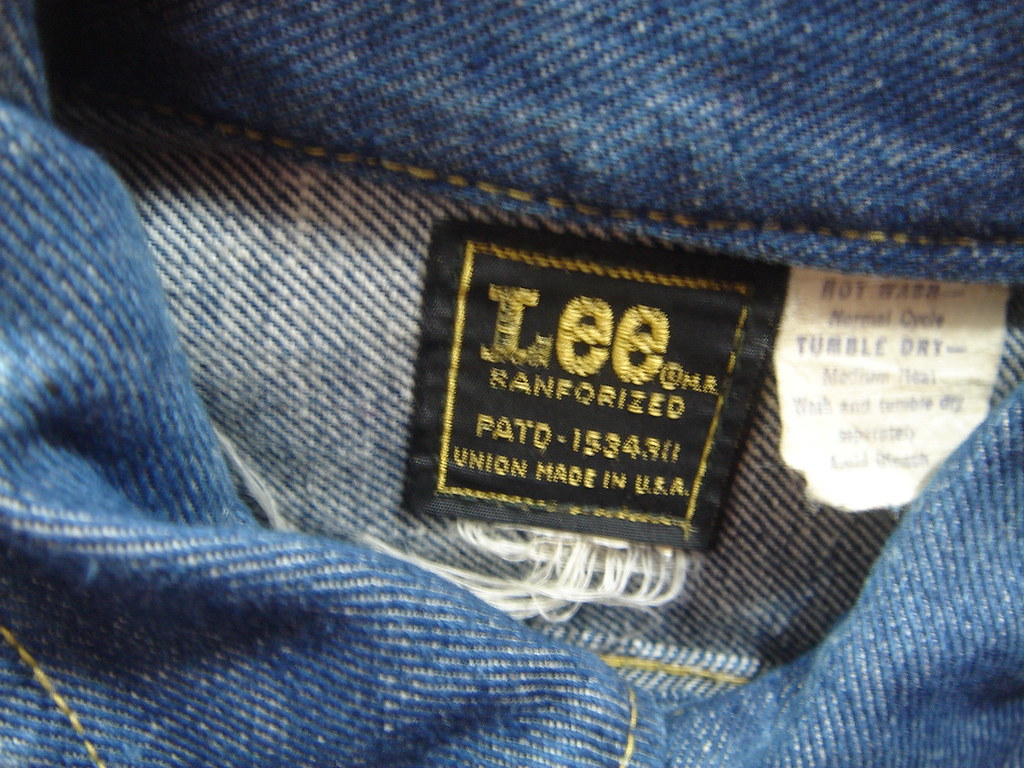This image is a detailed close-up of the inside tag of a blue denim garment, potentially a pair of vintage jeans or a jean jacket. The tag reads "Lee Sanforized" and includes additional details such as "Union Made in USA" and a possible model number "15343U." The specific type of clothing item is not immediately identifiable due to the hidden button. However, the classic blue denim fabric and the vintage appearance of the label provide a nostalgic touch, reminiscent of traditional American denim craftsmanship.